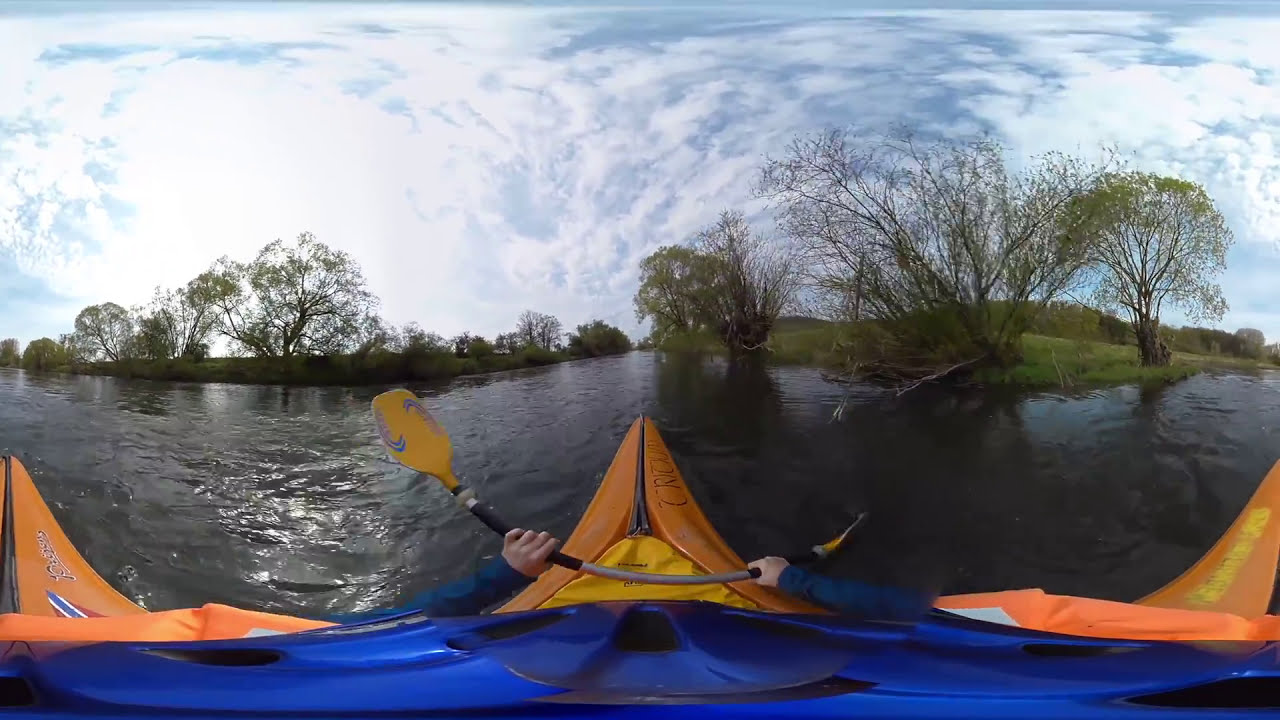This photograph offers a distinctive first-person perspective from the seat of a kayak, prominently showcasing the kayaker's hands gripping an orange swirled paddle, likely captured using a GoPro camera mounted on their head. The kayaker appears to be wearing a blue coat or shirt, and their forearms are visible in the image's center. Stretching out ahead is the front of the kayak, predominantly orange with yellow highlights, and partially legible black text reading "C-R-O" on its side. The kayak glides over dark, grayish water, surrounded by patches of grass and trees on either side. The trees, possibly willows, are in varying stages of leafing out, with some displaying light green new growth while others remain sparse. Above, the sky is a mix of blue, gray, and white hues, filled with scattered clouds, indicative of a mid-day outdoor setting. The entire scene is slightly curved, suggesting the use of a fisheye lens, offering a wide-angle view of the tranquil yet dynamic environment.